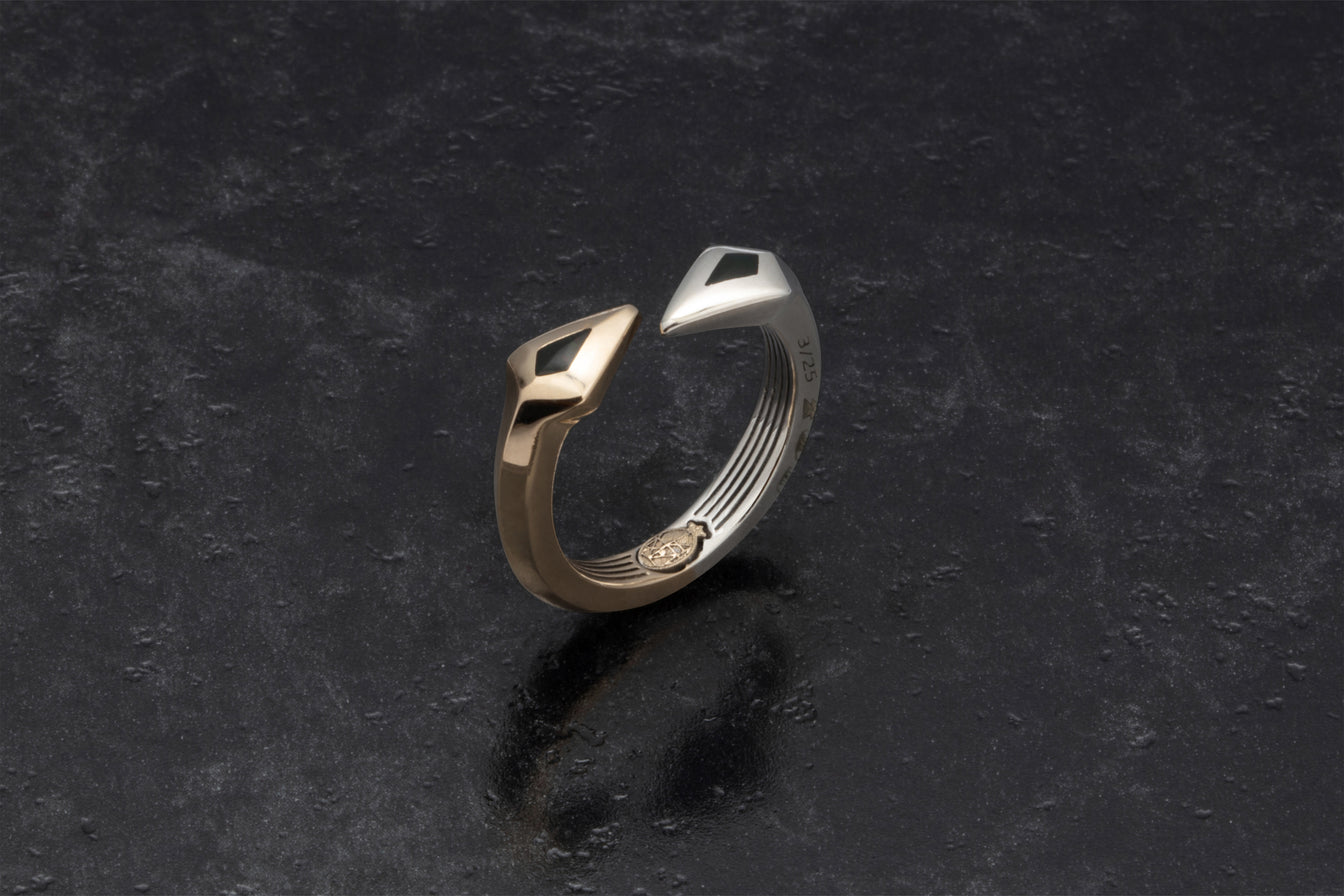This image is a professionally staged, full-color photograph taken indoors with artificial lighting. The setting is a textured dark gray or black countertop, which features noticeable textural bumps that would be palpable to the touch. Centered on this countertop is a ring, meticulously crafted from two types of metals: one a silver or platinum shade and the other a gold or bronze hue. 

The design is intricate, with the two metals meeting in the center in a striking pattern resembling snake heads, each adorned with a black diamond. The ring's 'heads' are positioned as if facing each other but do not touch, adding to the abstract aesthetic. The craftsmanship is further emphasized by a stamped emblem where the metals converge, indicating the artist's mark. 

A reflection of the ring can be clearly seen on the glossy countertop, reinforcing the ring’s placement. While the flawless appearance of the ring makes it seem as if it could be a digitally rendered image, this could also be attributed to the professional staging and possible digital enhancement to remove any standing supports, especially since the ring seems to levitate due to the angled design suggesting such alterations.